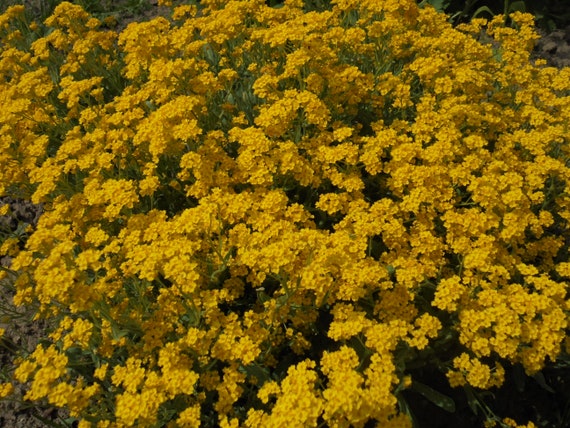The image depicts a detailed and close-up view of a sprawling, vibrant cluster of tiny yellow flowers, appearing almost like a professional photograph. The flowers are densely packed, forming hundreds of cheerful yellow blooms that mostly dominate the scene. Each flower showcases a cluster of bright yellow petals surrounding a slightly darker yellow center, often with hints of orange. The flowers are gathered in small bunches, each comprising around ten blooms, reminiscent of clusters seen on an azalea bush. Interspersed with the flowers are green leaves and stems, adding a fresh contrast to the image.

The lighting in the photograph is particularly well-balanced, highlighting the stunning saturation of the yellow petals, albeit with some areas being slightly out of focus. Additional details include a touch of brown and white within the flowers, lending a touch of natural depth. The lower right corner of the image is characterized by a denser, darker green than the rest of the scene, while the upper right corner appears slightly shadowed, giving some of the flowers a subtle brownish tint. The image distinctly lacks any presence of animals, people, other types of plants, or text, contributing to its clean and focused composition. The overall symmetry and vibrancy of the photo suggest an almost digital perfection, though it remains a pure photograph capturing the essence of a mesmerizing floral display.